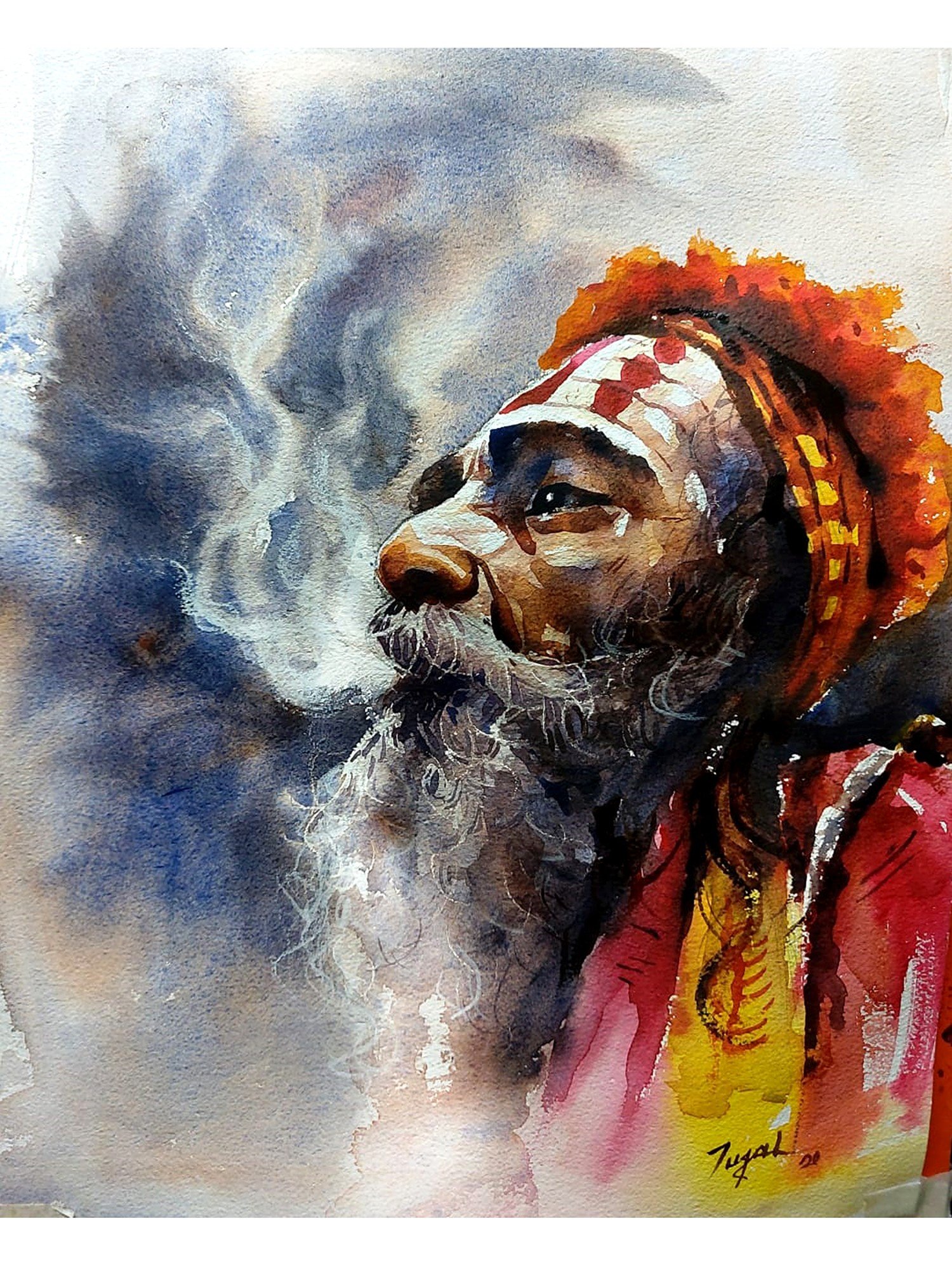This painting portrays an older man with a contemplative expression, gazing off to the left at a slight angle. The man has a long, gray beard that adds to his wise and weathered appearance. A cloud of smoke billows from his mouth, suggesting he is in mid-puff. His hair, tinged with shades of orange, is complemented by an orange and yellow headband, giving him a striking, colorful presence. Intriguingly, his forehead is adorned with a pattern of white and red splotches of paint. He is dressed in a loose-fitting red shirt that features a yellow band across it, adorned with an abstract, intricate pattern. In the lower right corner of the painting, the artist has marked their signature and a date, both of which are indistinct. The overall composition and vibrant colors evoke a sense of depth and character in the subject depicted.